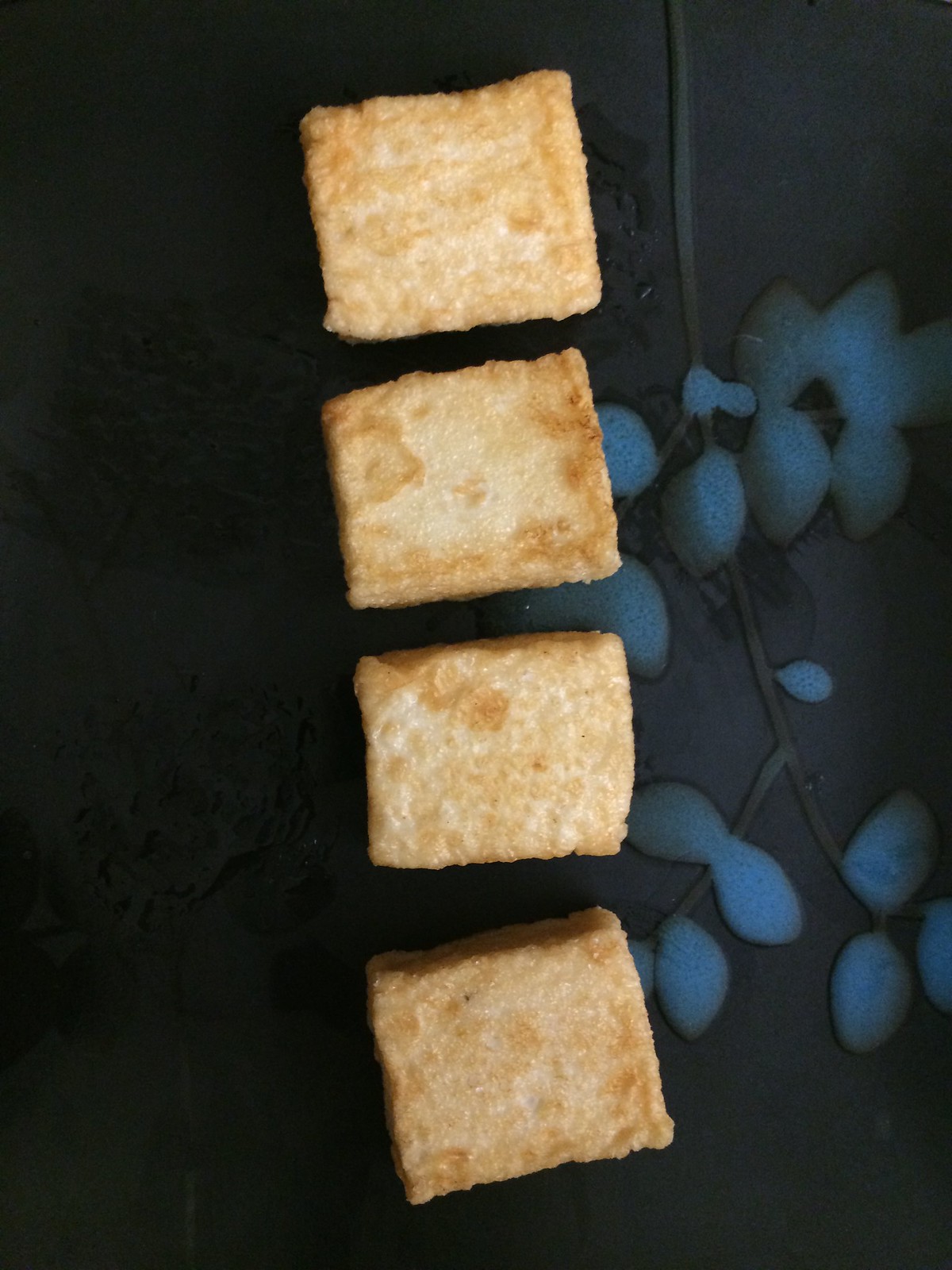The image showcases four uniform, golden-brown square cubes, each resembling croutons or tiny blocks of fried tofu, lined up vertically from top to bottom. These cubes, which have a texture and appearance somewhat like Cinnamon Toast Crunch, seem to be hovering against a dark, blurry background. The background is minimally lit and features shadowy, green, leaf-like elements—perhaps suggesting plants or a floral pattern often found on a tablecloth or pillow. The overall scene is somewhat unclear but gives the impression that the cubes are either suspended or carefully positioned to give a floating illusion. The nature of the background and the exact identity of the cubes remain ambiguous, adding a peculiar and mysterious quality to the photograph.